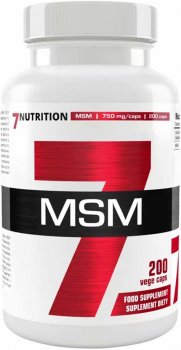A single white jar, prominently featuring the label for an MSM (Methylsulfonylmethane) supplement, stands against a neutral background. On the front of the jar, the letters "MSM" are boldly displayed atop a horizontal black banner that appears to wrap around the entire jar. Dominating the label is a large, bold red number seven, occupying a significant portion of the label space. Above the number, in smaller print, the text "Seven Nutrition" is clearly visible, indicating the brand. The jar also lists the quantity of the supplement, marked as "200 veggie caps" in red on the lower right section of the label. The designation "Food Supplement" is clearly printed underneath. The milligram dosage is mentioned but is partially obscured, making it difficult to read. Overall, the label is vibrant and eye-catching with important details prominently displayed.